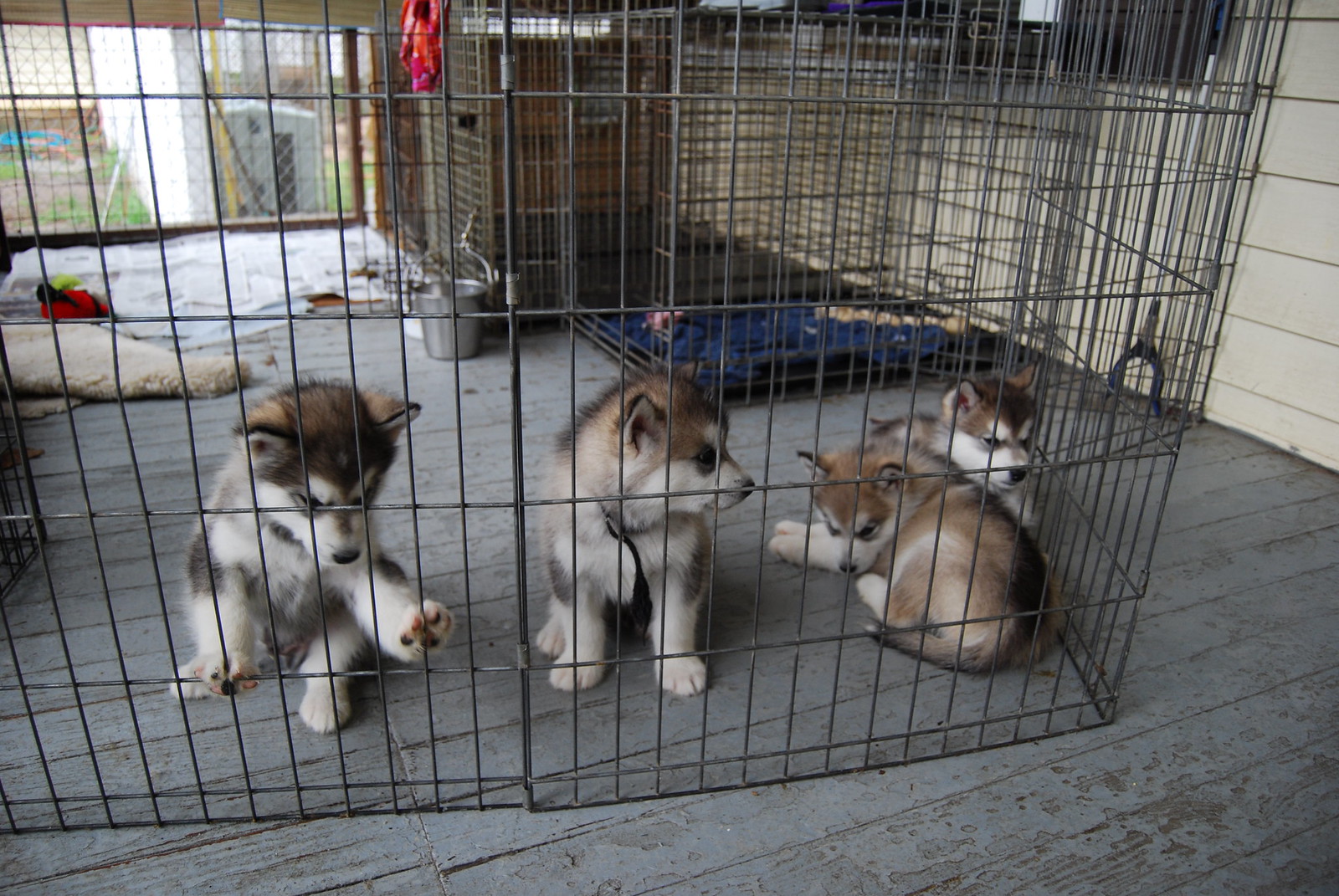In the photograph, there are four Siberian Husky puppies nestled inside a small wire cage situated on a wooden floor with a gray-brown tint. Each puppy exhibits unique yet similar features: they have fur that is a mix of white, gray, and brown, with a distinct dark brown “widow's peak” marking between their eyes and white muzzles. Some of the pups have white tips on their tails, while others' tips are black. All of the puppies appear to be around eight weeks old, with ears that stand upright in a triangular shape.

One puppy has its paw resting on the cage, while another lounges in a cuddled position beside a sitting sibling. The fourth puppy sits on its front paws in the middle, its head turned to the right. None of the puppies are directly gazing at the camera, adding a natural and candid element to the image. Two of the puppies on the left are sitting up on their hind legs, while the two on the right are reclining on all fours.

In the background, several items are visible: there is a play mat, a potential dog bed inside another cage, and a metal pail for water. An adjacent wooden wall and a window overlooking the backyard lend a homey atmosphere to the setting, complemented by a hint of a doghouse visible outside. This detailed scene encapsulates the tender and playful environment of the young husky puppies.